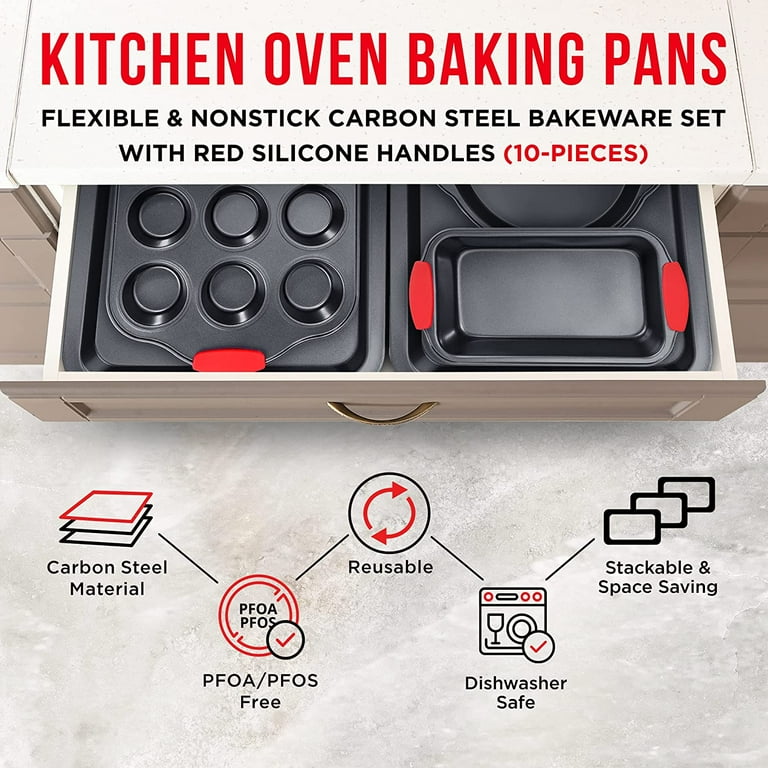This image showcases an advertisement for a kitchen oven baking pan set. At the top, in bold red letters, the text reads "Kitchen Oven Baking Pans." Below that, it describes the set as a "Flexible and Nonstick Carbon Steel Bakeware Set with Red Silicone Handles, 10 Pieces." The image features an open brown cabinet and drawer, displaying part of this 10-piece set: a visible cupcake tin, bread pan, and a partial view of a pie tin, all in black with distinctive red silicone handles. The background features a marble floor. Overlay text from left to right labels the bakeware's features: "Carbon Steel Material," "PFOA/PFOS Free" indicated by a circle with arrows pointing to the terms, a "Reusable" symbol moving upward, "Dishwasher Safe" with a downward arrow pointing to a dishwasher icon, and three squares labeled "Stackable and Space-Saving." Together, these elements highlight the practical and durable qualities of this versatile, nonstick bakeware set.